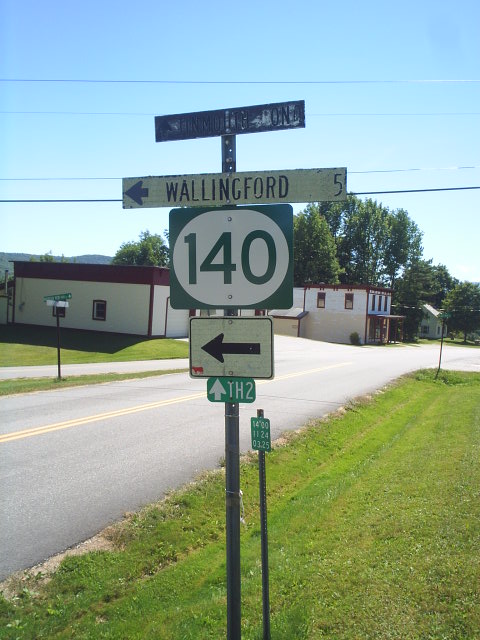The image depicts an outdoor scene under a clear blue sky transitioning to white at the horizon. Dominated by a mountain in the distant background, the scene moves forward to a mixed treeline featuring different types of trees—some tall and full, others shorter but similarly lush. Below the treeline, a significant, elongated white building with a brown top and a square front section with an awning stands prominently. In the foreground, a grassy area runs alongside a two-lane road with yellow center lines. The road is bordered by a sidewalk and is dotted with several street signs.

A series of signs detail the directions: prominently displayed is a white sign with black lettering and an arrow pointing left that says “Wallingford 5.” Below it, a green sign features the number 140 and a left-pointing arrow, followed by another sign indicating TH2 with an upward arrow. The roadway and signs suggest a locale rich with greenery and structured with clear directional cues, hinting at a small town or neighborhood setting. Another segment of the road is visible on the left, reinforcing the structured yet tranquil environment captured in the photograph.